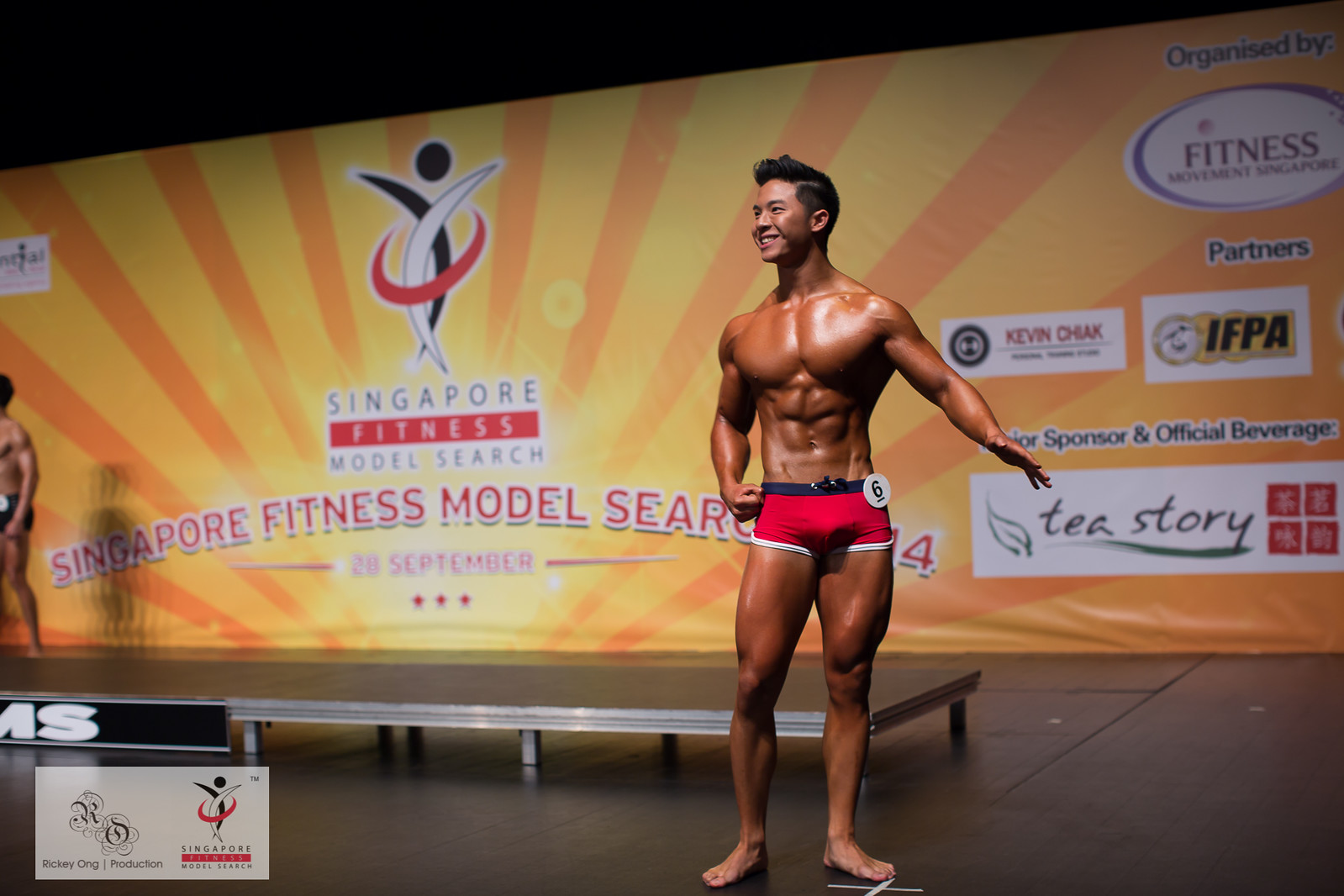In this vibrant photograph from the Singapore Fitness Model Search event, a muscular fitness model takes center stage, adorned in tight red pants with white and dark blue stripes at the upper and lower portions. The model, who appears to be of Asian descent, sports well-groomed black hair and beams a wide, confident smile. Behind him, the professional event's black stage contrasts against a radiant yellow and gold backdrop featuring multiple logos on the right. Dominating the backdrop is a bold logo with the text "Singapore Fitness Model Search," framed by a bright sunburst effect. Interestingly, the backdrop also hints at the event date, "28th September," although partially obscured by the model. To the left, partially cut off, is a glimpse of another contestant's left arm and leg. The entire scene captures the intense yet celebratory atmosphere of the fitness model competition.